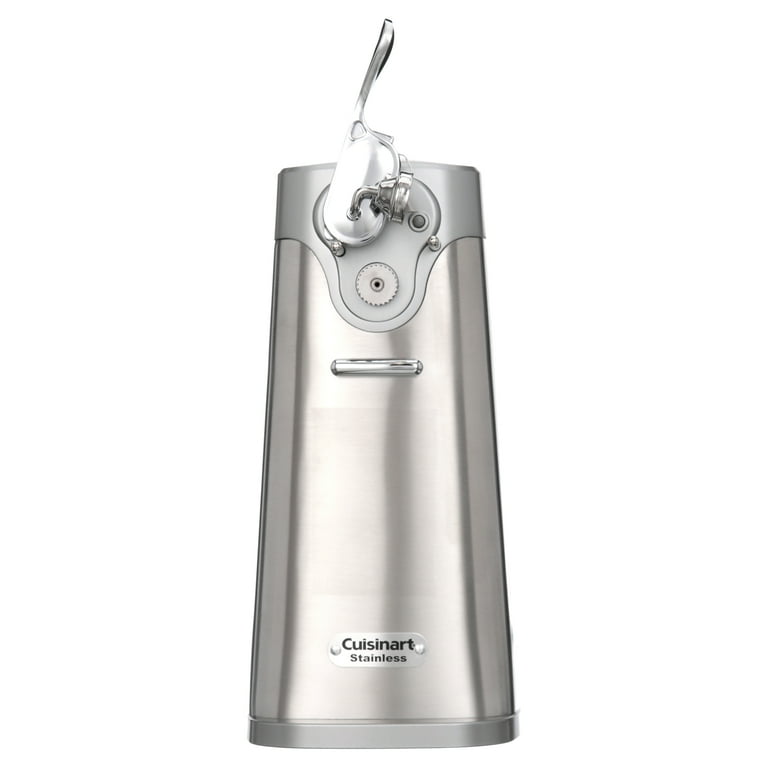This is a promotional photo showcasing a Cuisinart stainless steel electric can opener in a detailed front view. The can opener stands approximately six inches tall with a base around three inches wide, tapering slightly to two inches at the top, giving it a cylinder-like shape. The entire structure is made of solid stainless steel, featuring a shiny yet brushed finish. Towards the bottom of the can opener, there's a small metal plaque that reads "Cuisinart Stainless," secured by two rivets on either side. The can opening mechanism sits at the top, comprising a traditional design where you position the can underneath the cutting wheel, lower the handle, and the attached magnet secures the lid. This mechanism is in a slightly different hue of stainless steel, adding a subtle contrast. The can opener appears robust and well-crafted, designed to be functional and aesthetically pleasing, though no background or table is visible in the image.